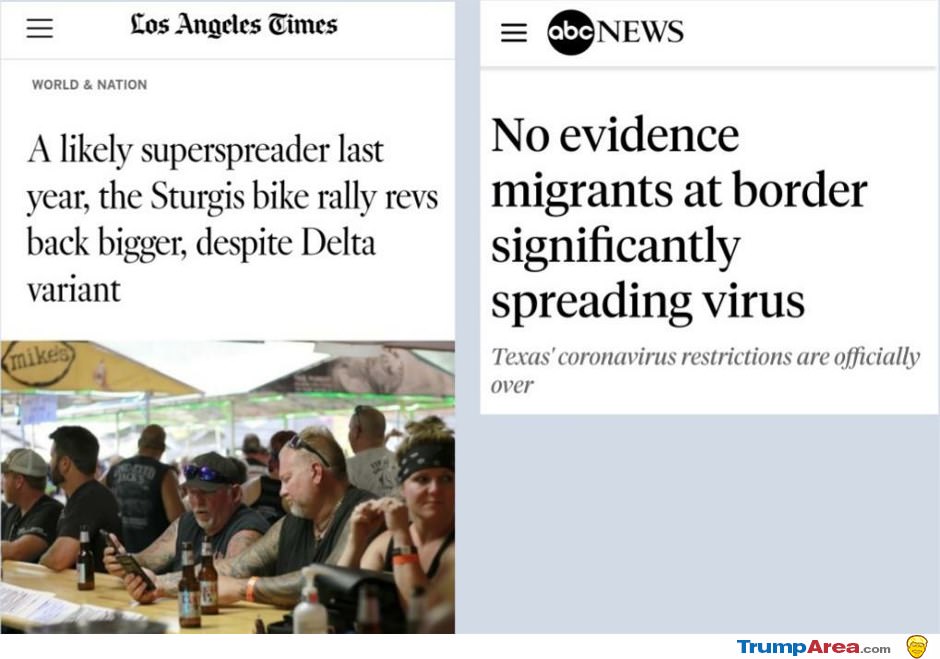The image is a composite of news story screenshots with a gray background, presented in a wide rectangular format. In the bottom right corner, "TrumpArea.com" is displayed. The phrase "Trump" is highlighted in blue, while "Area" is highlighted in red. 

The left side of the image features a headline from the L.A. Times under the "World & Nation" section, occupying the entire height of the rectangle. The headline reads: "A likely super spreader last year, the Sturgis Bike Rally revs back bigger despite Delta variant." This story refers to the annual Sturgis Bike Rally in South Dakota, a well-known event for Harley-Davidson motorcycle enthusiasts from across the country.

On the right side of the image is a news headline from ABC News, contained within a white box that extends about two-thirds down the canvas. The headline states: "No evidence migrants at border significantly spreading virus. Texas' coronavirus restrictions are officially over." 

Both headlines are from the COVID-19 era, highlighting how scientific issues became politicized. The surrounding context and the association with "TrumpArea.com" appear incongruent with the subjects of the headlines, which both support scientific viewpoints.